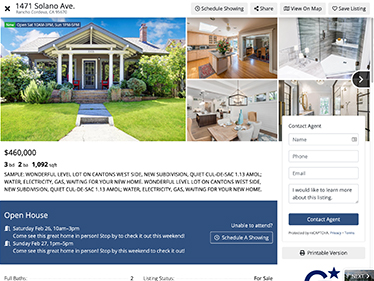Detailed Caption: 

This image depicts a real estate listing for a house located at 1471 Solano Avenue. The listing price is prominently displayed at $46,000. Although the exact dimensions are difficult to discern due to the poor quality of the image, it mentions the property is 1,192 square feet and includes three bedrooms and two bathrooms.

The central part of the image showcases a main photo of the house, accompanied by four smaller thumbnail images beneath it for different views of the property. An icon to the right of these thumbnails indicates more photos can be viewed.

To the upper right of the images, there are four buttons arranged vertically. The buttons read as follows: the first is unclear, the second appears to be a share button, the third is for viewing the location on a map, and the final one is likely for saving the listing.

Further to the right is a contact form for potential buyers. It includes fields for entering a name, an email address, and an option to request more information. Below this, a blue contact agent button is visible.

At the bottom left to the center of the image, a blue rectangle denotes information about an open house, with "Open House" written in white text. The specific details about the open house are unclear, but it suggests it might be scheduled for Sunday, possibly from 10:00 AM to 3:00 PM.